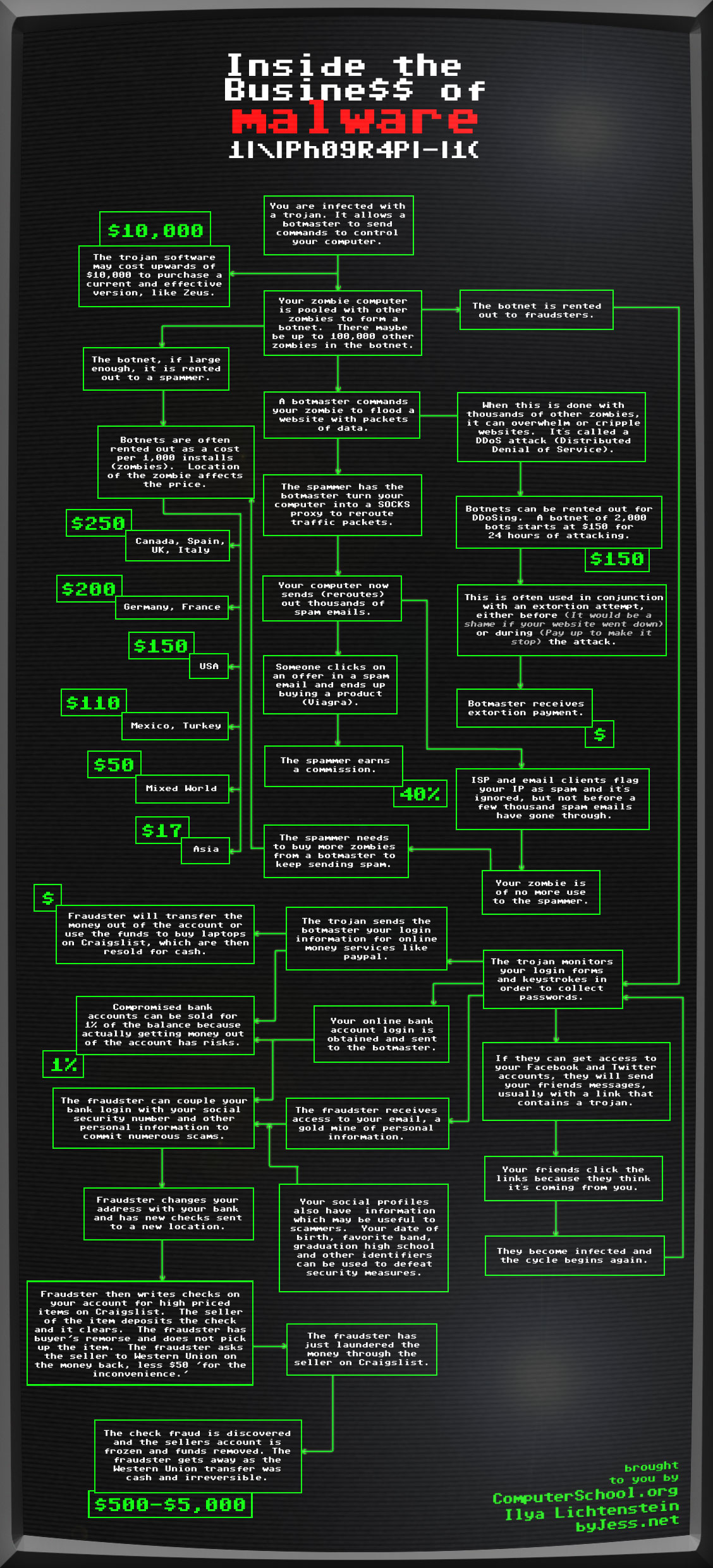Caption: 

This detailed flowchart, titled "Inside the Business of Malware," uses a stark visual presentation to illustrate the financial impact and inner workings of malware attacks. The title is prominently displayed, with the word "Malware" in larger, bold red letters, making it stand out against the otherwise white text. Below the title, the flowchart features a series of interconnected steps, all presented on a black background. The steps and various annotations are written in white lettering, while significant errors and inflection points are highlighted in bright green, drawing attention to critical parts of the process. Each box in the flowchart contains tiny, fine-print text, making specific details difficult to read without close inspection. Key financial figures such as $10,000, $250, $200, $150, $10, $50, $17, 1%, 40%, and $500 to $50,000 are surrounded by dollar signs to emphasize the monetary stakes involved. Notably, a portion of the text reads, "You are infected with a Trojan. It allows a blaster to command control of your computer," underscoring potential vulnerabilities. At the bottom, the flowchart is credited to "Computerschool.org," with a bright green callout stating "A live lesson by Jess.net" positioned in the bottom right-hand corner. The intricate, densely packed information within this flowchart serves as a robust educational resource, potentially aimed at showcasing the threats and financial consequences of malware.